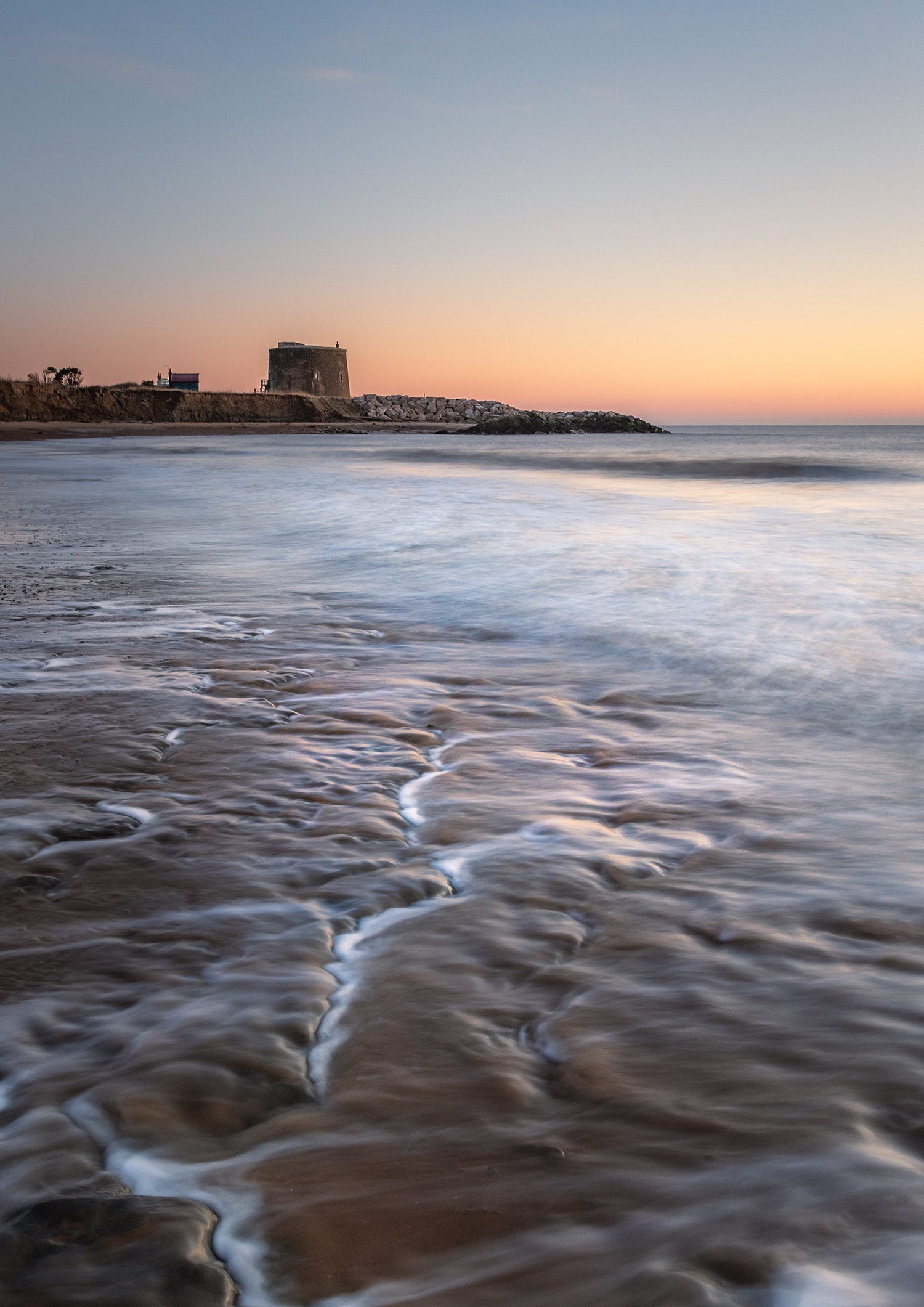The photograph captures a tranquil coastal scene at dawn, bathed in the soft hues of a rising sun with yellows, oranges, and pinks blending into a gradually lightening blue sky. The main focus of the image is the serene waves gently gliding across the sandy shore, creating delicate bumps and ridges rather than high crests. In the backdrop stands a small, rectangular stone building, possibly the base of an old lighthouse, flanked by other smaller structures. This building sits atop a light brown landmass fortified with a rocky protective barrier to shield it from the encroaching sea. The overall composition evokes the timeless beauty of coastal mornings, highlighted by the gentle interplay of light and water.